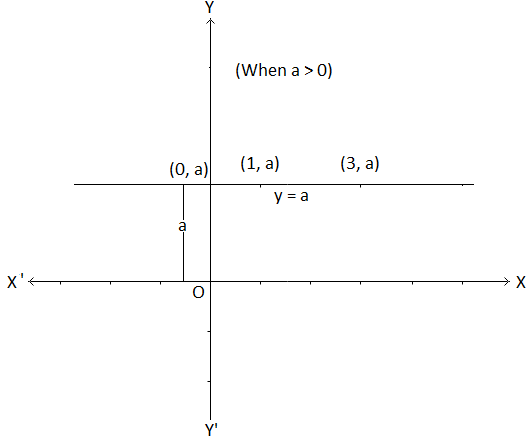The black and white image illustrates a mathematical Cartesian graph with clear coordinates and labeling. The y-axis runs vertically with an arrow pointing upwards, marked with 'y' at the top and 'y-prime' at the bottom. The x-axis runs horizontally with arrows at both ends, labeled 'x-prime' on the left and 'x' on the right. At the intersection of the axes is the origin labeled 'O'. 

In the image, there is a horizontal line above the x-axis, which is annotated with specific coordinates: starting from the left, it reads (0, a), followed by (1, a) and further right, (3, a). These points are indicated with brackets and are placed along this horizontal line. Below this line, it is noted that \( y = a \), symbolizing the y-value for each coordinate point on this line. Above the line, there's an annotation reading "when \( a > 0 \)". The image also displays regular hash marks along the x-axis and the y-axis, emphasizing the graph's increments and structure.